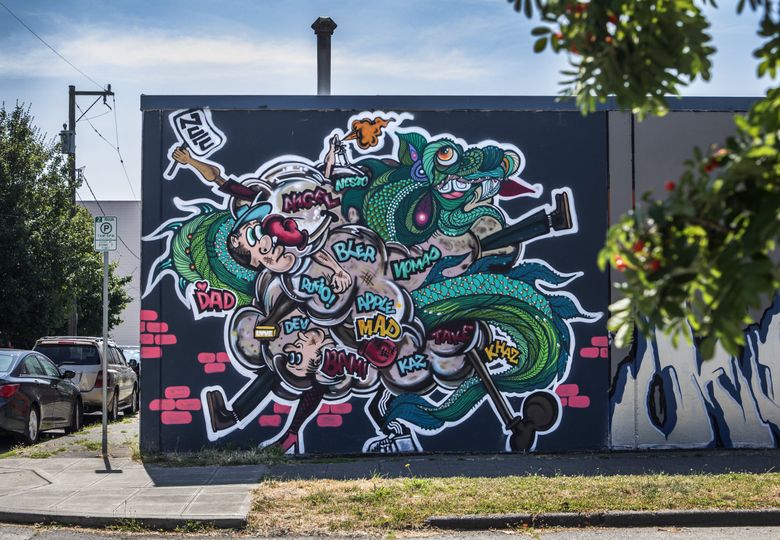The photograph captures the side of a building adorned with a vibrant graffiti mural on a black and dark gray background. The lower half of the wall features painted red bricks. Dominating the chaotic and dynamic scene is a green, serpentine creature that resembles an octopus intertwined with a dragon, complete with big eyes and emitting smoke-like gray puffs. Interspersed within the writhing forms are human heads and disembodied arms and legs, one of which holds a sign reading “Zulu.” Scattered throughout the mural are various names and words such as “Dad” (with a heart above it), “Miguel,” “Nomad,” “Apple,” “Mad,” “Kaz” (spelled differently in various spots), “Blur,” “Dev,” “Rukio,” “Blair,” and “Bam.” The mural extends into a neighboring graffiti image on a gray background, partially obscured by branches. In front of the wall is a sidewalk and some ragged grass, with a "No Parking" sign visible. The street on the left side of the mural has several parked cars.